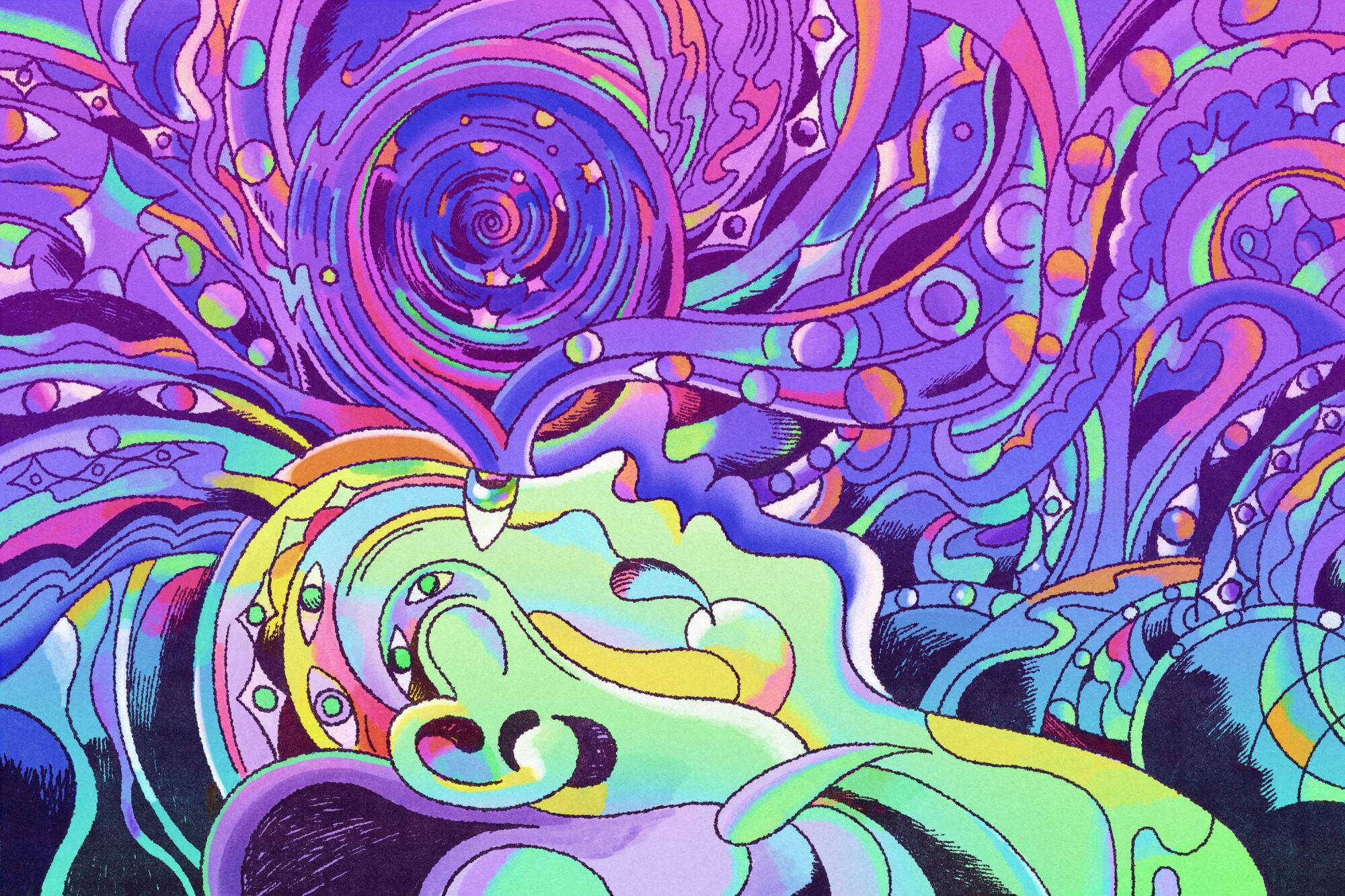This vibrant and psychedelic art piece features an abstract figure, potentially a person or alien, reclining with their head resting on a pillow-like form. Dominated by various purple hues in the background, the image is a swirl of bright colors including greens, pinks, oranges, yellows, blues, and whites. The central figure, primarily green with hints of purple, displays multiple eyes—six in total—and a single ear positioned unconventionally. The eyes and swirling shapes seem to emanate from the figure’s mouth, adding to the surreal and abstract nature of the scene. The background is filled with intricate circular patterns and long, border-like lines, reminiscent of octopus tentacles. The overall effect is that of a highly detailed and colorful tapestry, with a mesmerizing flow of shapes and colors that evoke a psychedelic experience.